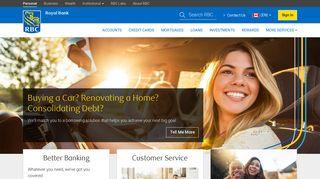**Screenshot Analysis of Financial Services Website**

The screenshot features a website highlighting financial services, adorned with a multi-colored design and specific call-to-actions for users. The website's layout includes:

1. **Header**: 
   - A top section with a black rectangle followed by a blue strip, then transitioning into a white background.
   
2. **Sign-In Functionality**:
   - Located at the top right, a yellow rectangle bearing the text "Sign In" in black allows users to log in.

3. **Main Content Area**:
   - A large, albeit slightly blurry, image of a smiling woman driving a car is prominently displayed. She appears cheerful with her teeth visible.
   - Overlaid on the image is a text prompt with important financial questions: "Buying a car?", "Buying a home?", "Considering debt?", and "Consolidating debt?".
   - Below these questions, there is a call-to-action button labelled "Tell Me More."
   
4. **Additional Sections**:
   - Directly beneath the main image are three distinct squares:
     - The first square features an image of what appears to be a couple, a woman and a man.
     - The second square contains an icon or text related to "Better Banking."
     - The third square highlights "Customer Service" offerings.

5. **Navigation**:
   - A search bar is included, aiding users in quick navigation.

This descriptive portrayal encapsulates the essence of the website, emphasizing its user-focused financial solutions and clear navigational pathways.